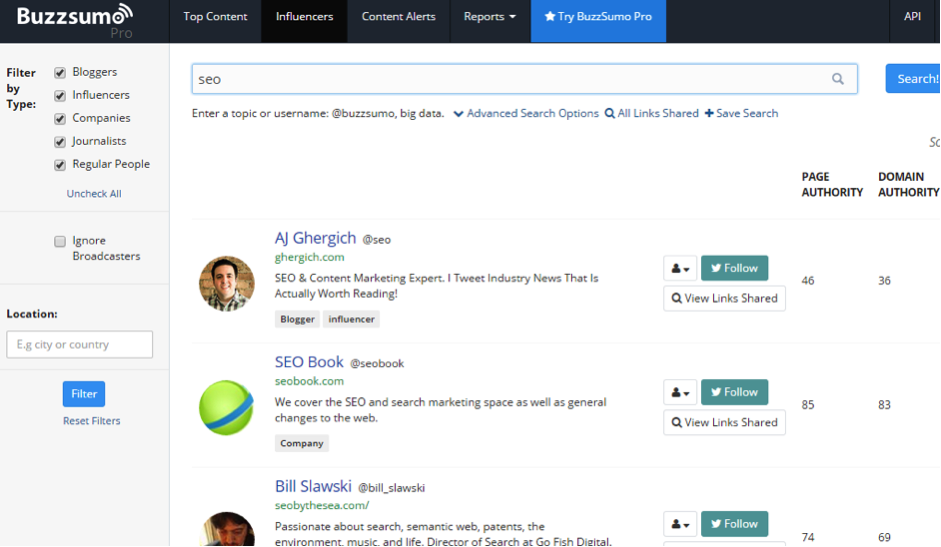This image is a detailed desktop screenshot of the BuzzSumo Pro platform in use. The operating system, web browser, and web address are not visible, but the interface reveals an extensive array of options and search capabilities. At the top, there is a black menu bar with white text displaying the BuzzSumo logo, where the "O" resembles a donut emitting Wi-Fi signals. The menu includes options like "Top Content," "Influencers," "Content Alerts," "Reports," and a blue button labeled "Try BuzzSumo Pro," marked by a white star. To the right, the menu shows “API.”

On the left, a filtering panel offers various options for refinement, including content types like bloggers, influencers, companies, journalists, and regular people, all currently selected. The panel includes an "Uncheck All" option and an "Ignore Broadcasters" checkbox, which is not selected. Users can filter by "Location," specifying city and country, with "Filter" and "Reset Filters" buttons available.

Centered in the interface is a search bar with the query "SEO" entered. Adjacent to it is a blue "Search" button. The interface suggests search capabilities like "Enter a topic or username at BuzzSumo," "big data," and "advanced search options." Below this, options like "All links shared" and "Save Search" are visible.

Search results display profiles of various influencers and entities related to SEO:

1. **AJ Ghergich** (@SEO) - Described as an SEO and content marketing expert, AJ Ghergich tweets industry news worth reading. Tagged as a blogger and influencer, his profile includes options to interact via Twitter and view shared links. His page authority is 46, and domain authority is 36.

2. **SEO Book** (@seobook.com) - This company covers SEO and search marketing, along with general web changes. Interaction options include following and viewing shared links. Its page authority is 85, and domain authority is 83.

3. **Bill Slawski** (@Bill_Slawski) - Known for his passion for search, the semantic web, patents, environment, music, and life, Bill Slawski is the Director of Search at Go Fish Digital. His profile shows a page authority of 74 and a domain authority of 69.

The screenshot effectively portrays how BuzzSumo Pro enables users to find and filter various types of content providers and influencers related to specific topics.